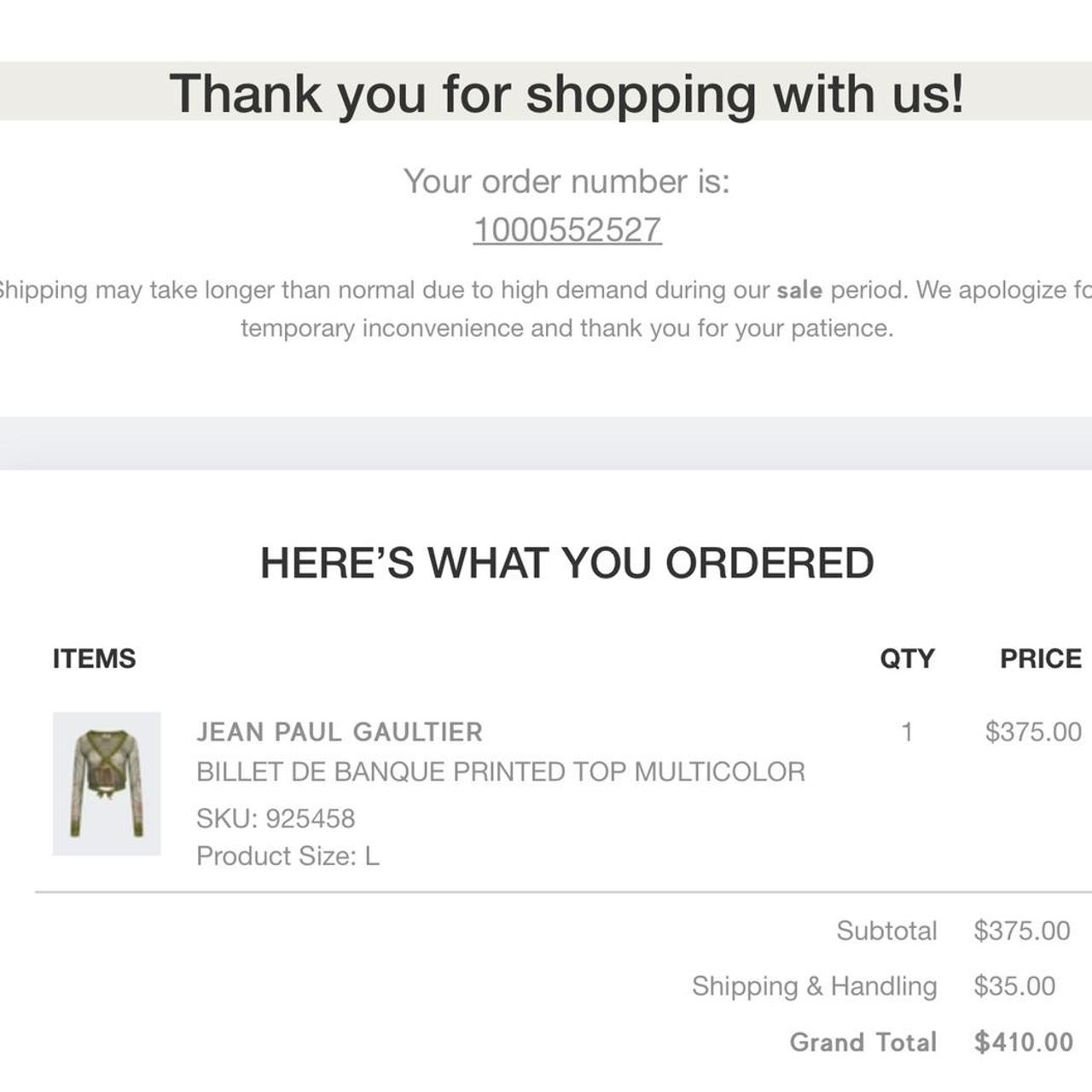At the top of the image, there is a confirmation screen from an e-commerce site set on a peach-colored background strip, featuring black letters. The message reads, "Thank you for shopping with us!" Beneath that, in centered gray text, it says, "Your order number is:", followed by an underlined order number "1-00-552-527" on a new line. Below the order number, a message states, "Shipping may take longer than normal due to high demand during our SALE period. We apologize for the temporary inconvenience and thank you for your patience." However, the left and right edges of this message are slightly trimmed, cutting off parts of the letters "S" in "Shipping" and "R" in "for."

Following this, another peach-colored field is visible before transitioning to a white background. On this white section, in bold capitalized text, it reads, "HERE'S WHAT YOU ORDERED." The listed item is "Jean-Paul Gaultier Belay de Banque Printed Top - Multicolor" with SKU "925458" and size "Large." An image of the item, described as a low v-neck long sleeve top, is placed under the item description. Beneath it, the order details specify a quantity of "1" and a price of "$375." A thin gray line separates these details from the subtotal, which also reads "$375." Below this, shipping and handling costs "$35," leading to a bolded grand total of "$410."

The last line of text reads, "So enjoy your top, I guess." The top is described as potentially being a mix of gray, brown, and olive colors.